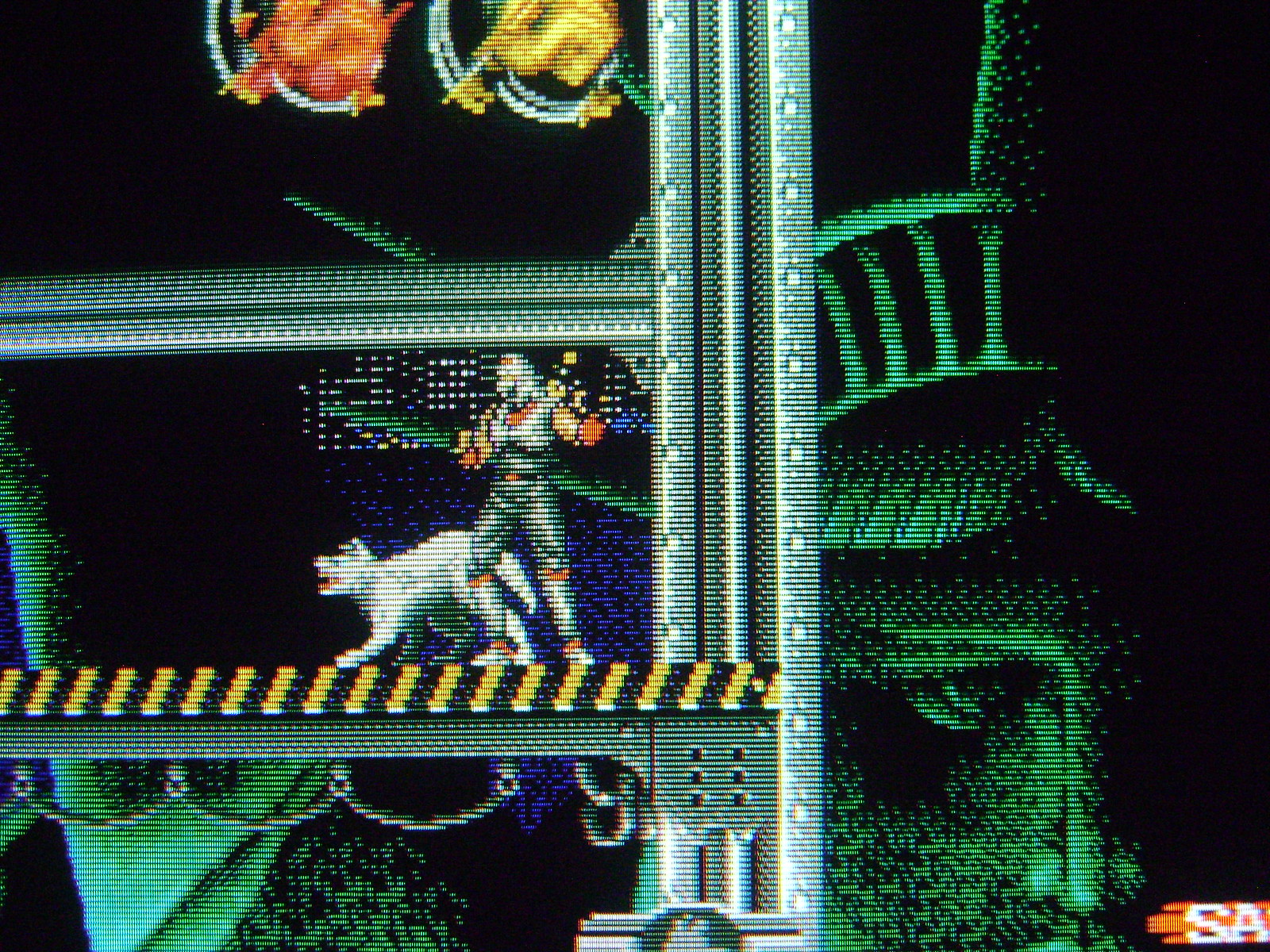A pixelated screenshot from an unidentified video game showcasing a scene set against a predominantly black backdrop with contrasting green structures and splashes of yellow, red, and black elements. At the center of the image stands a humanoid character in armor, potentially armed, though it's unclear from the image. Beside the character is a dog, and both are facing the same direction, possibly indicating anticipation or alertness. No opponents are visible in the scene. In the bottom right corner, the letters "S" and "A" are displayed, though their significance remains ambiguous, possibly representing the player's initials or part of the game’s branding.